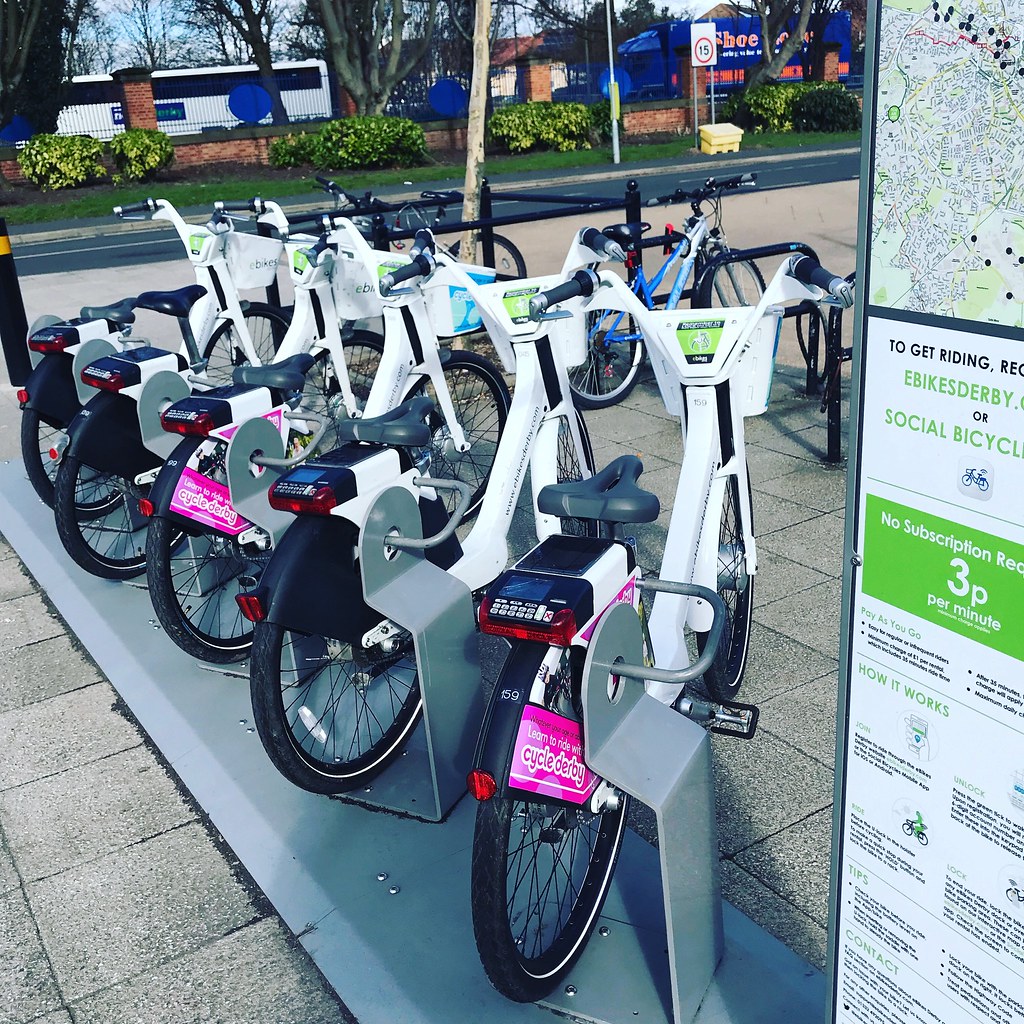The image features a close-up of a public bike rental station with five white e-bikes, all equipped with black seats, neatly locked into a metal stanchion. These self-service bikes are ready for renting and pedaling around the city. The bikes are parked on a stone walkway composed of concrete or stone tiles. To the right of the station, there is a detailed map of the city along with information regarding rental procedures and pricing. In the background, a street scene unfolds with a white bus and a large tractor trailer passing by. Across the street, there is a lush, grassy area adorned with bushes, behind which a brick wall and fencing can be spotted. Beyond the fence line, a line of trees is visible, emphasizing the sunny, blue sky overhead. Additionally, a yellow sign indicating a speed limit of 15 miles per hour can be seen in the vicinity.